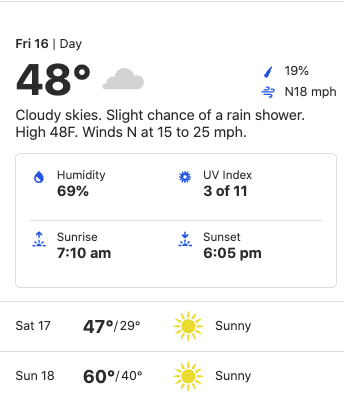Screenshot with a white background displaying a detailed weather forecast:

- **Friday, FRI 16**: 
  - **Current Temperature**: 48°F
  - **Condition**: Cloudy with a slight chance of rain showers
  - **Icons**: Cloud, Raindrop
  - **Precipitation Probability**: 19%
  - **Wind**: N at 18 MPH
  - **Detailed Forecast**: 
    - High: 48°F
    - Winds: 15 to 25 MPH
    - Humidity: 69%
    - UV Index: 3 out of 11
    - Sunrise: 7:10 AM
    - Sunset: 6:05 PM

- **Saturday, SAT 17**: 
  - **Temperature**: 47°F / 29°F
  - **Condition**: Sunny
  - **Icon**: Sun

- **Sunday, 18**: 
  - **Temperature**: 60°F / 40°F
  - **Condition**: Sunny
  - **Icon**: Sun